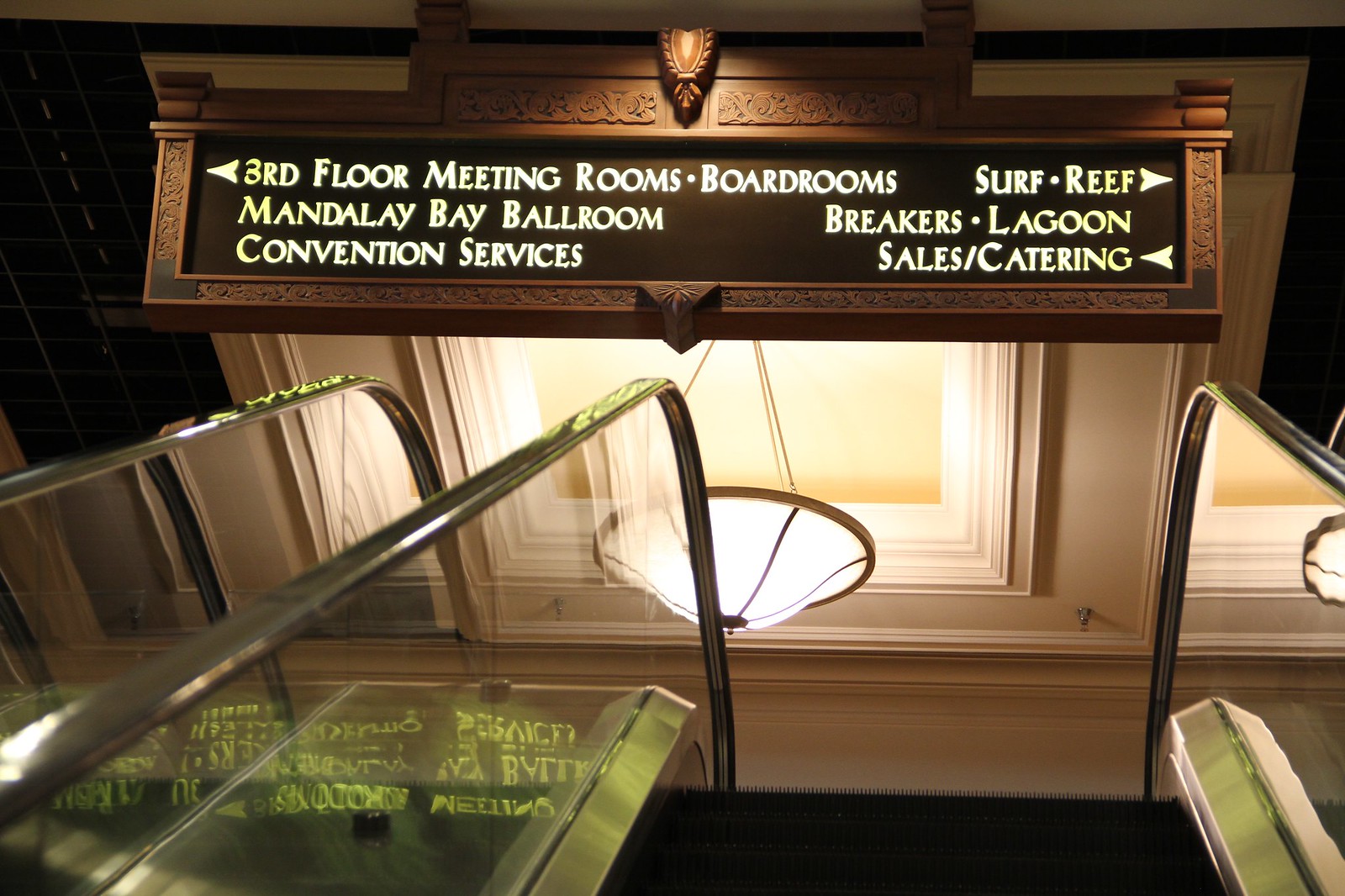The photograph depicts the interior of the Mandalay Bay Ballroom, specifically focusing on a set of central escalators, with silver railings and glass panels, that transport guests between floors. Prominently displayed above the escalators is an ornate brown sign with white text, enclosed in a wooden frame, pointing towards different facilities within the building. The sign details various destinations such as "third floor meeting rooms," "boardrooms," "surf and reef," "breakers lagoon," "sales/catering," and "convention services," with directional arrows indicating their locations. The ceiling, adorned with brown and white trim, features yellow-hued light fixtures that illuminate the space, reinforcing the grandeur and meticulous design of this indoor casino setting.